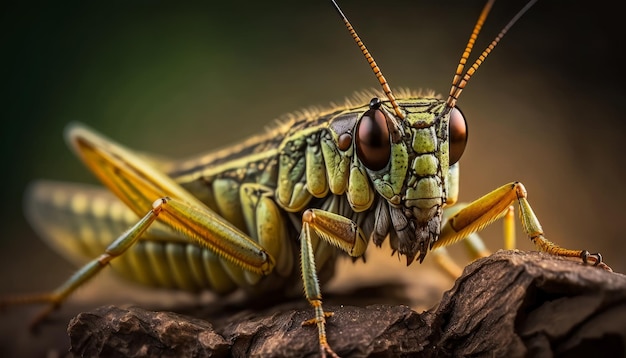This close-up, high-quality macro photograph captures an incredibly detailed view of a green cricket in a natural setting. The focus is on the cricket's head and the left side of its body, showcasing its intricate features. The cricket's head boasts two large, distinct eyes, predominantly described as red or brown, and three prominent spikes. Its antennae, brown with stripes, extend outward, adding to the creature's striking appearance. The cricket's body displays a range of green shades with some yellow tints, and the fine hairs on its legs are clearly visible. The insect is perched on a brown rock or piece of wood, though the exact surroundings are heavily blurred, emphasizing the cricket's form. The macro perspective makes it appear as though the cricket is staring directly at the camera, dominating the entire frame with its detailed, lifelike presence.